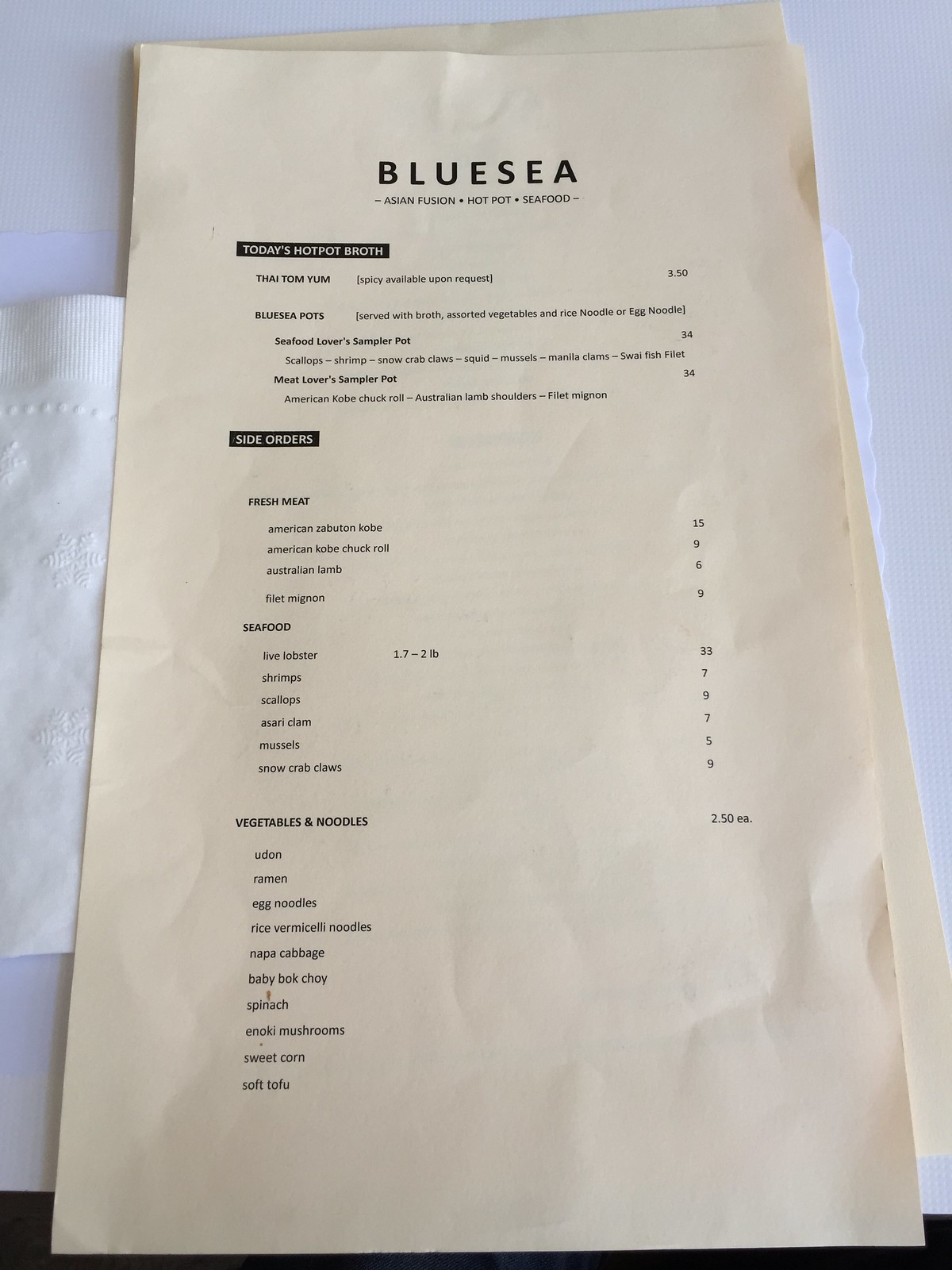A detailed miniature menu rests on a pristine, white surface. The paper is delicately placed atop a napkin, which is partially visible, extending from the left-hand side. The napkin is adorned with subtle floral designs and features decorative dots along its edges and lines on its ridge, adding a touch of elegance. Beneath the menu, a second piece of paper, identical in size and design, peeks out slightly from the top and right sides.

The menu itself bears the title "Blue Sea" at the top, followed by the description "Asian Fusion, Hot Pot, and Seafood," each phrase separated by a small black dot. Below this introduction, a black rectangle announces "Today's Hot Pot Bra." Two options are listed beneath this heading, with their corresponding prices listed to the right. Further down, another black rectangle introduces "Side Orders." This section is divided into three categories: Fresh Meat, Seafood, and Vegetables & Noodles. Each category contains a variety of selections with their respective prices detailed below.